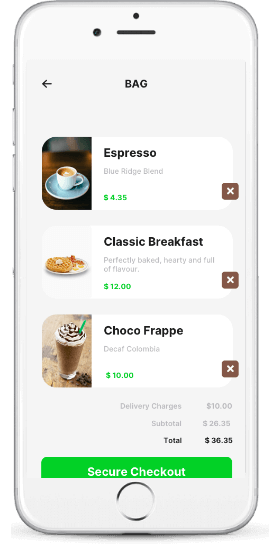This image showcases a white cell phone displaying a food ordering app. At the top of the screen, there is a black bar with a centrally positioned black dot above it, followed by a larger black dot and another smaller dot to its left. Below this, on the left-hand side, a black arrow is visible. Dominating the center of the screen are the bold, uppercase letters "BAG" written in large black font. 

Further down, there's an image of a coffee cup on the left side, featuring a white cup on a blue saucer placed on a brown table. Next to this image, the green text reads "Espresso, Blue Ridge Blend," priced at $4.34. On the right, there is a brown square icon with a white X inside.

Below that, an image of a waffle is displayed on the left side, presented on a white plate against a white background. Accompanying this image, the description reads "Classic Breakfast, perfectly baked, hearty, and full of flavor," priced at $12.00 in green text. To the right, there's another brown square box with a white X.

Beneath this section, there's a picture of a chocolate frappe in a glass with a straw, topped with whipped cream and drizzled with chocolate, placed on a brown table. Next to this image, the green text spells out "Choco Frappe, Decaf Columbia," priced at $10.00. On the right, there's yet another brown square box with a white X.

Following this, the delivery charges are listed as $10.00. The subtotal is shown as $26.35, bringing the total to $36.35.

At the bottom of the screen, there is a green button labeled "Secure Checkout."